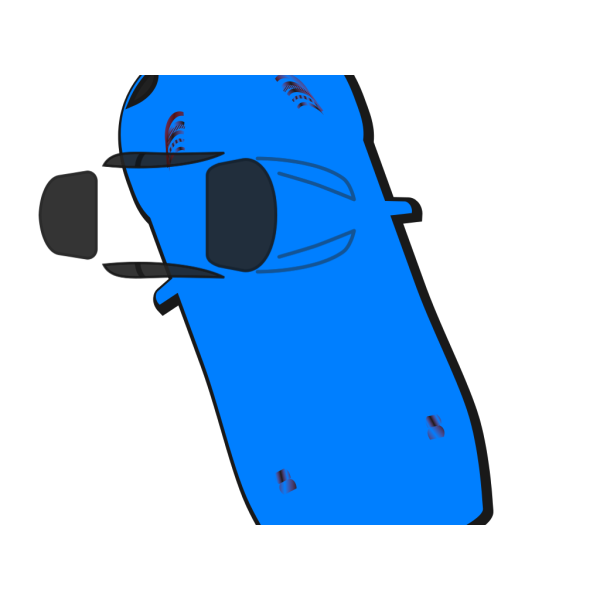The image depicts a blue, oval-shaped vehicle viewed from a bird's-eye perspective, featuring both digital and hand-drawn elements. The primary blue vehicle is elongated and slightly tilted to the left, characterized by black windows and protruding black front headlights on the top left. Additionally, small black rearview mirrors are present on both the left and right sides. The windshield and back windshield appear misplaced, adding to the impression that this could be a customizable design interface.

Overlaying the larger blue vehicle is a black-outlined depiction of another smaller vehicle, aligned to the right. This superimposed vehicle features elements that resemble facial features, such as eyes, a mustache, and brows, arranged in an anthropomorphic manner. These elements include black eyebrows positioned at the top right and left, and eyes and a mustache below on the top left, giving the impression of a face emerging from the abstract design. The overall composition remains unfinished and seems like a whimsical digital creation blending automotive design with human-like characteristics.